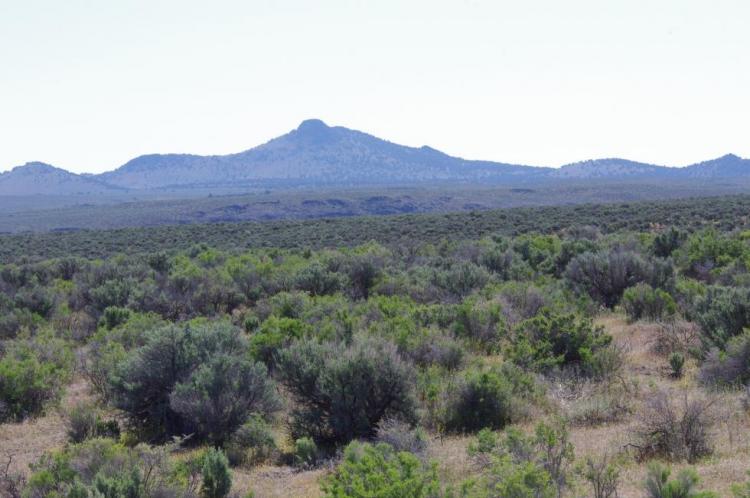In this horizontally elongated, vintage photograph, the viewer is presented with a low-resolution image marked by slightly muted colors, evoking an aged and nostalgic aesthetic. The scene captures a desert landscape juxtaposed against a backdrop of low-lying, jagged mountains or canyons. The bottom half of the image is dominated by a desert terrain, characterized by a primarily brownish expanse dotted with sparse vegetation, including low-lying trees and bushes varying in shades from light green to dark, almost teal. The sky above is a pale whitish hue, devoid of the typical blue vibrancy, suggesting either an overcast atmosphere or the effects of age on the photograph. On the horizon, the mountainous terrain stretches from left to right, its jagged silhouette softened by distance and possibly the same types of vegetation seen in the foreground, although the exact details are obscured by the photograph's color discoloration. This daylight scene is devoid of any human presence, highlighting the stark, quiet beauty of this seemingly untouched desert landscape.